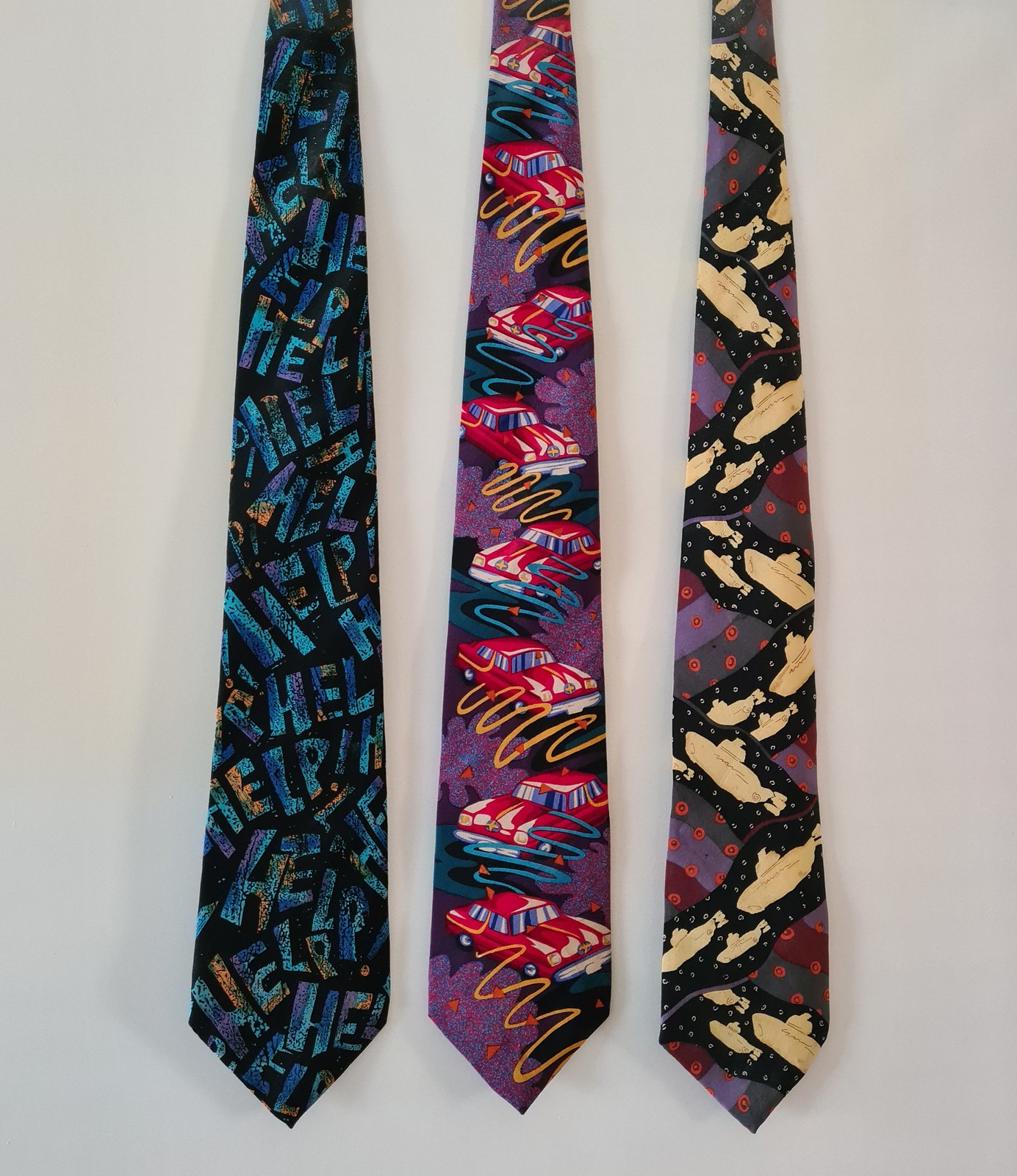Against a light blue background, three stylish neckties hang in a row. The tie on the left is black, adorned with the word "HELP" repetitively printed in abstract blue lettering. The middle tie features a dynamic design of shiny red cars with white illuminated highlights, driving amidst yellow swirly lines, set against a background of pinkish-purple floral patterns. The final tie on the right is distinguished by geometric triangles in shades of gray, purple, and red along the sides. Down the middle, yellow submarines swim through an imaginative black space filled with white circles and dots. Each tie is of equal width and displayed in full length, emphasizing their unique, bold patterns.